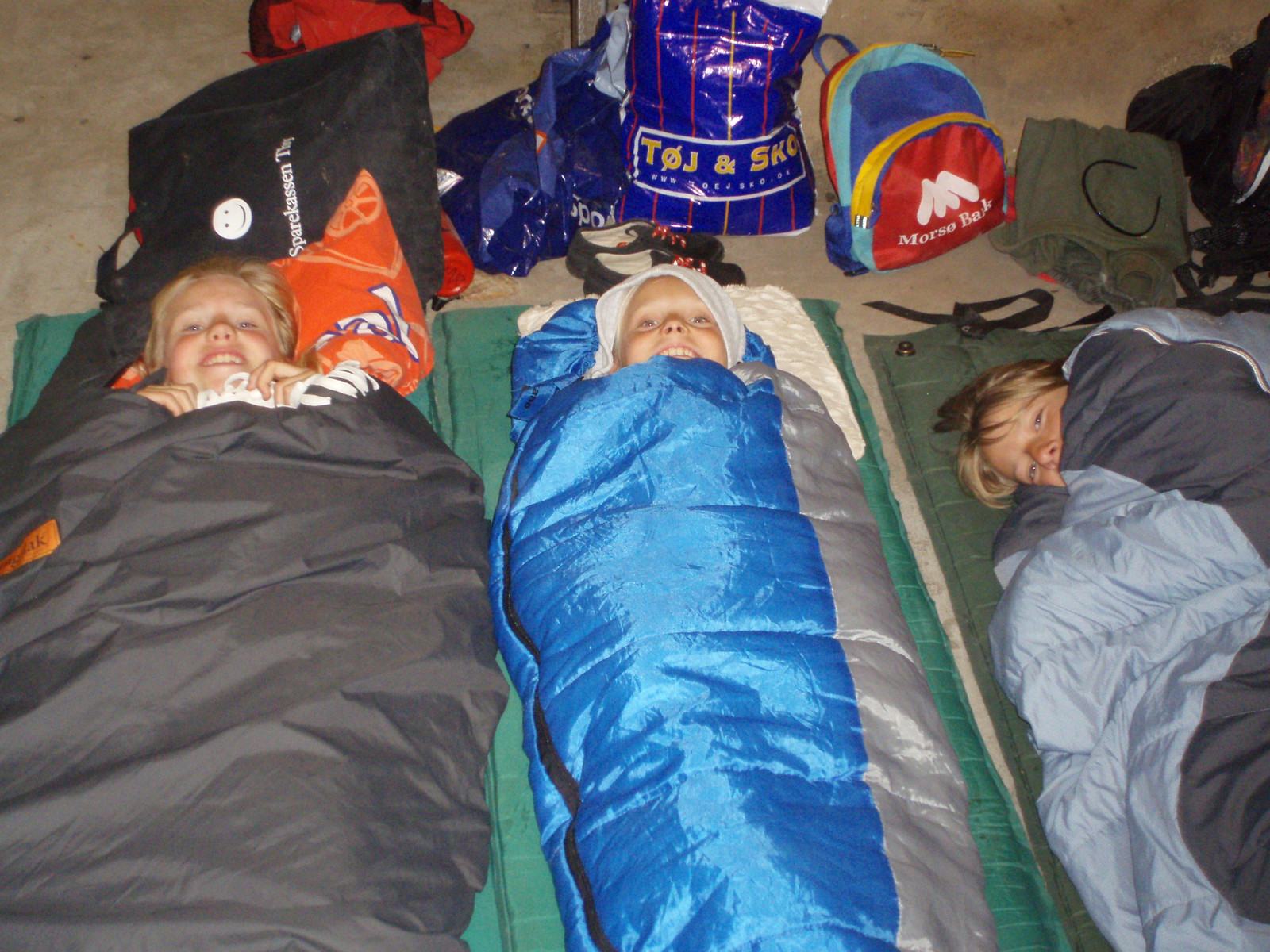In this detailed image, we see three boys, possibly around eight or nine years old, lying in sleeping bags on green air mattress pads, likely at a sleepover or a makeshift indoor camping setup. All three boys are awake and looking at the camera, with two of them smiling broadly with open mouths, suggesting they are enjoying their adventure. Each boy is nestled in a different colored sleeping bag: the child on the left is in a gray sleeping bag with an orange pillow under his head and a black bag positioned behind him. The middle child is using a shiny blue and gray sleeping bag, which seems to include a hoodie, and his face is angled upwards giving an almost up-the-nose view. Behind him is a blue plastic bag with red and yellow stripes, marked with the letters "T-O-J" and "S-K-O", along with a small multi-colored backpack in red, yellow, blue, and turquoise. The boy on the right is in a gray and darker gray sleeping bag, lying on a green pad, and has an army green pile of clothes with a headband on top behind him, as well as a black bag to his right. The backdrop includes a beige indoor-outdoor carpet and heaps of luggage, backpacks, and shopping bags making the indoor setting blur the line between a cozy room and an adventurous campout.